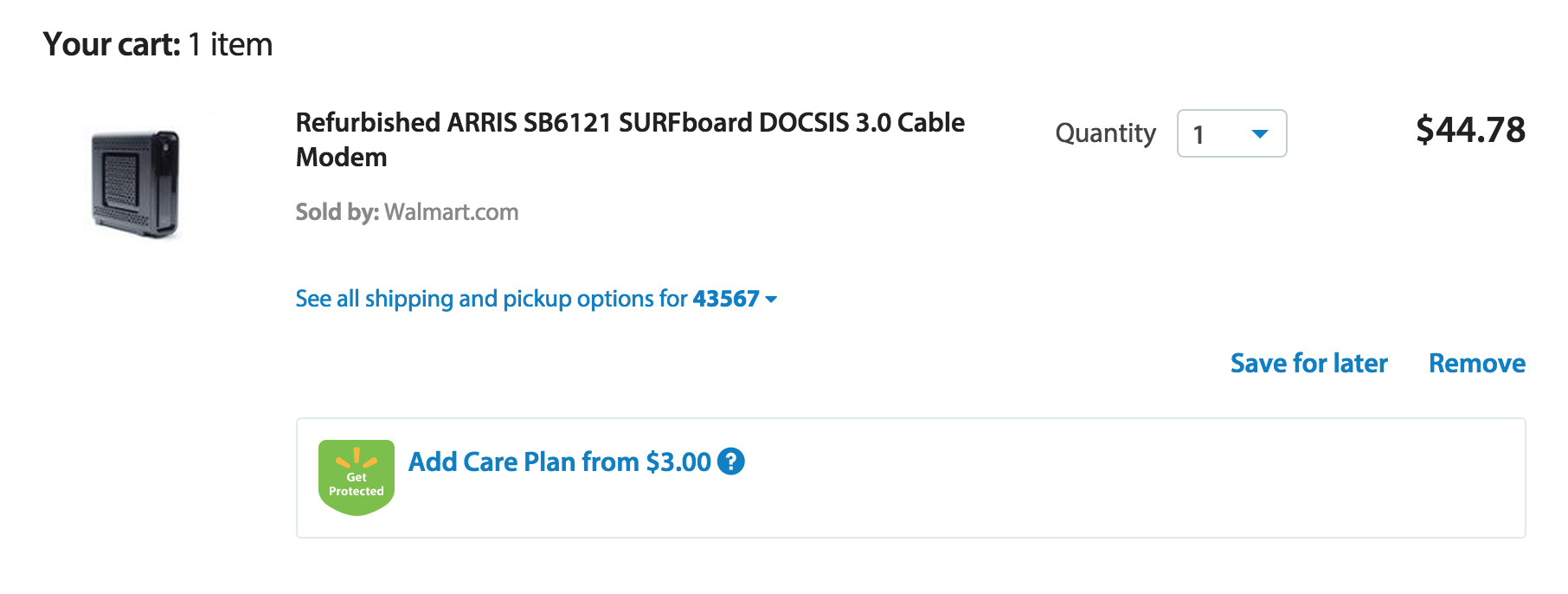The webpage features a predominantly white background, displaying a shopping cart interface. At the top left corner, bold black letters announce "Your Cart" followed by "One Item" in regular font. Below, there is an image of a sleek, black modem with visible vents on its sides.

To the right of the modem image, in smaller bold black letters, is the product description: "Refurbished Arris SB6121 Surfboard DOCSIS 3.0 Cable Modem." Beneath the product title, additional details state "Sold by Walmart.com, Quantity: 1, Price: $44.78."

Further down, an option is presented in blue text: "See All Shipping and Pickup Options." Next, a total price of "$435.67" is mentioned, followed by links for "Save for Later" and "Remove" in blue.

At the bottom, a rectangular area showcases a green shield icon adorned with three yellow rays, symbolizing protection. Next to this icon, in blue letters, is the prompt: "Add Care Plan for $3," along with the message "Get Protected" in white text under the shield.